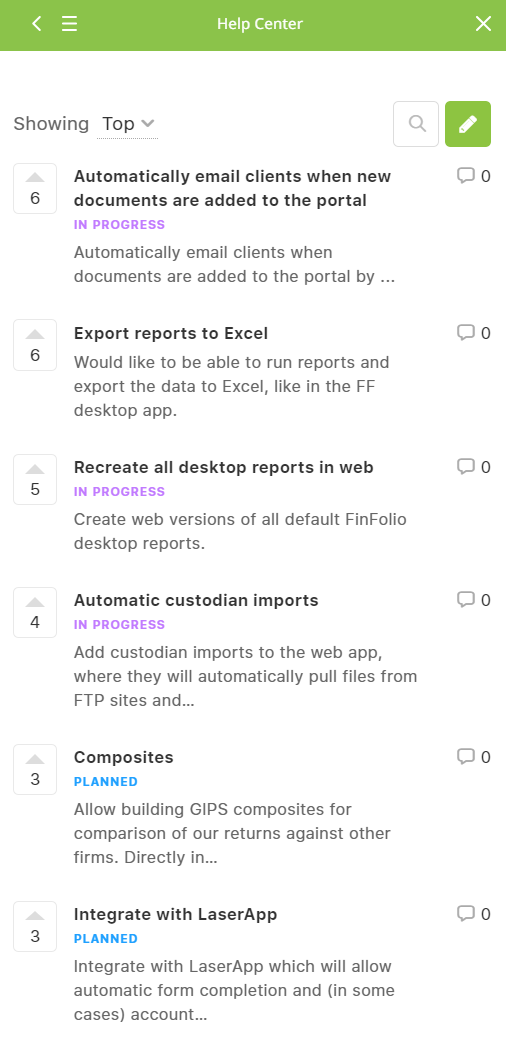The image displays a "Help Center" section of a website or app, prominently highlighted by a lime green banner at the top with the text "Help Center." Directly below, on the left side, it reads "Showing" followed by the word "Top" accompanied by a down arrow.

The section lists various tasks:
1. **Automatically email clients when new documents are added to the portal.**
   - Status: In Progress (purple)
2. **Export reports to Excel.**
   - Status: In Progress (purple)
3. **Recreate all desktop reports in web.**
   - Status: In Progress (purple)
4. **Automatic custodian imports.**
   - Status: In Progress (purple)
5. **Composites and integrate with laser app.**
   - Status: Planned (blue)
6. **[Another unspecified task]**
   - Status: Planned (blue)

On the left of each task, there are boxes with up arrows and numbers indicating priority or votes, with values listed sequentially as 6, 6, 5, 4, 3, and 3 from top to bottom. Additionally, there are small comment icons on the right side of each task, each displaying a count of 0.